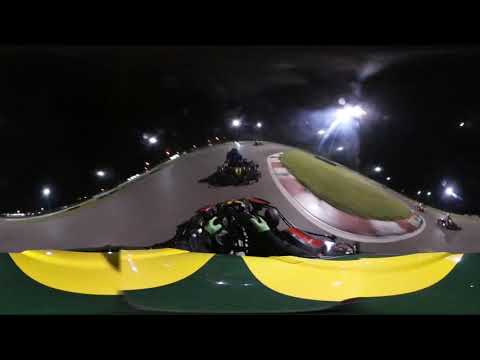This detailed caption combines elements from each voice description, emphasizing the shared and repeated observations:

This is a nighttime photograph of a go-kart race, possibly capturing a distorted 360-degree panoramic view. The scene is set against a black sky, indicating it's taken at night, with various bright white lights and street lamps illuminating the track and surroundings. In the foreground, from what appears to be a helmet-mounted perspective, we see a go-kart adorned with a green flag featuring yellow, banana-shaped markings. The racer in front is wearing a white helmet and a blue jacket, while the main driver in the shot sports lime green gloves and a distinctive helmet decorated with yellow circles. The go-karts are mostly dark black, racing on a gray track with red and black squares marking the corners. The grassy patch near the edge of the track ensures safety in case of a crash. Two additional go-karts follow behind in the background. Notably, there are no living people visible beyond the racers themselves, and the vividly painted details on the front go-kart resemble a green monster with yellow eyes. The overall image exudes a disorienting, almost artistic feel, potentially due to the panoramic distortion and varied light sources.